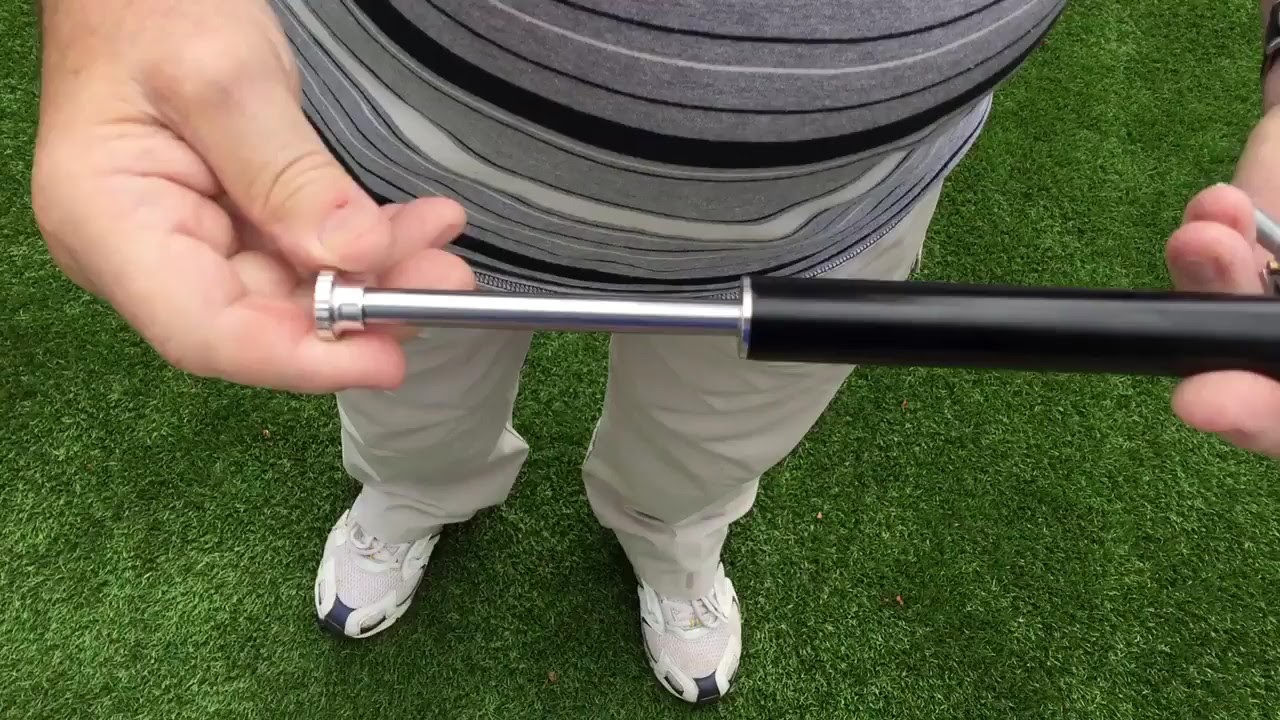The horizontally aligned rectangular image is a close-up view of a man's midsection and hands, set against neatly manicured, artificial green turf. The man, whose face is not visible, is dressed in white tennis shoes with black toe caps, beige khaki pants, and a horizontally striped shirt featuring gray, white, and black stripes. His right hand is prominently visible in the upper left corner, holding a device that extends toward his left hand, partially visible on the right side of the image. The device consists of a cylindrical black base with a slightly thicker diameter than the attached silver rod, which appears to be a bit shorter. The man seems to be demonstrating the tool, holding it delicately between his right thumb and index finger. The setting and his attire suggest that he is on a golf course or another type of athletic field.